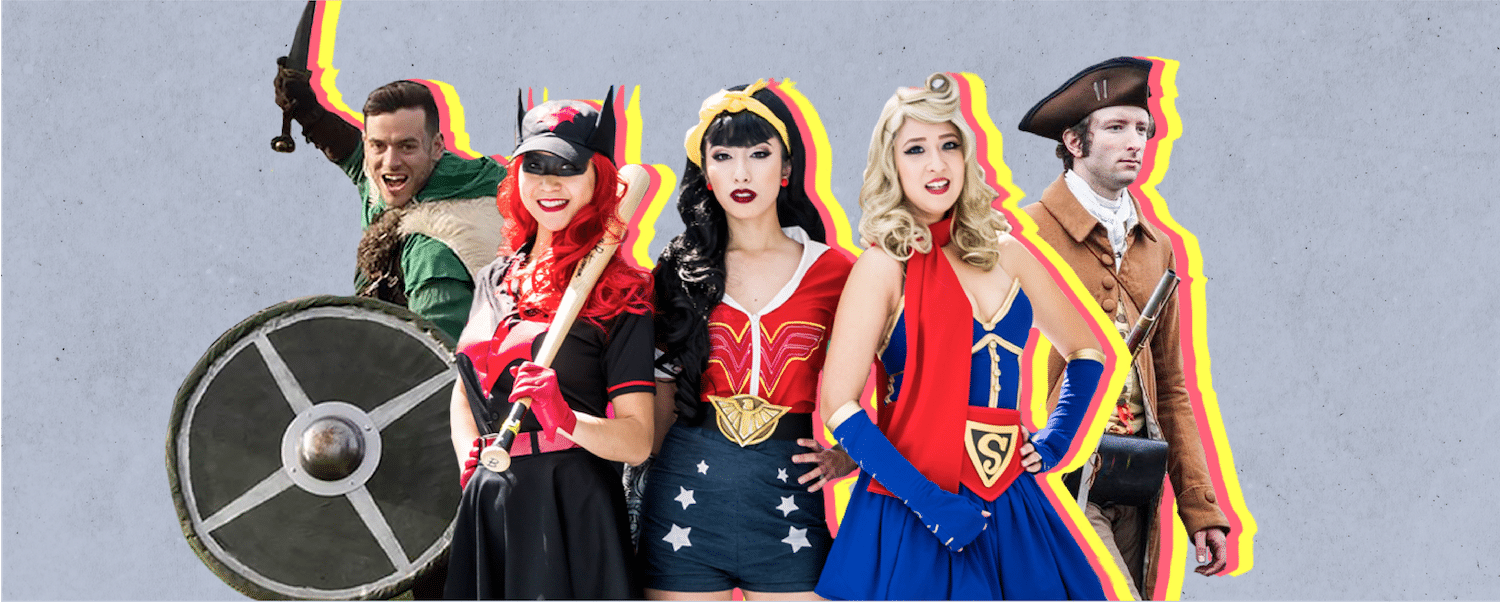In the image, five individuals, three women and two men, are dressed up in various elaborate costumes, hinting at a lively cosplay or Halloween gathering. The background is a simple gray, making their vibrant attire stand out. Each person is outlined with a decorative pink and yellow shadow, enhancing the festive feel.

On the far left stands a man with brown hair, donned in a green outfit paired with a fur coat, resembling a Viking warrior. He holds a circular shield with a metallic dome in the center and raises a sword high. Next to him, a woman with bright red hair is dressed like a baseball player, wearing a black domino mask and a baseball hat with large ears. She sports a black dress with red accents, holding a baseball bat over her shoulder.

In the center, a woman embodies Wonder Woman, with long black hair tied back by a yellow ribbon. She wears a red shirt emblazoned with a stylized 'W,' blue pants with white stars, and has striking black and red lipstick. To her right, another woman channels Supergirl, characterized by her long, curly blonde hair and a blue dress adorned with gold accents. Her outfit includes a golden 'S' belt and a red scarf draped around her neck.

On the far right, a man dressed as a colonial explorer from the 1700s completes the group. He wears a tan and brown colonial suit with a dark brown tricorn hat, facing to the right with an air of historical intrigue. All of them appear to be thoroughly enjoying themselves, adding to the cheerful and dynamic ambiance of the scene.